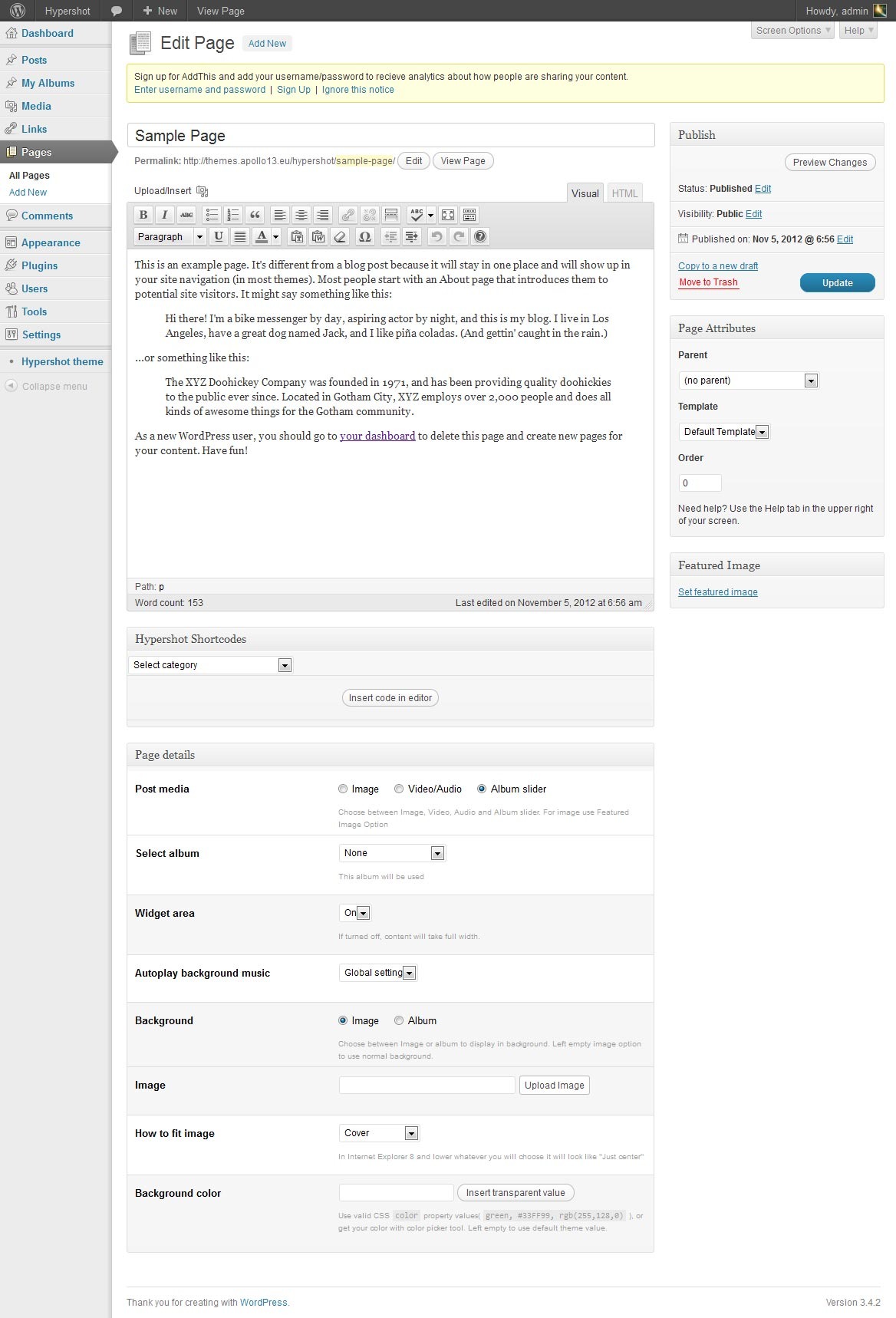Screenshot of a WordPress Web Page in Development

The image showcases a WordPress webpage under construction in a development environment. The screenshot, noticeably taller than it is wide, appears to be captured from a computer screen. 

At the very top sits a black toolbar featuring the WordPress logo on the left side. The title of the website, "HyperShot," is prominently displayed next to it. The browser view is centered on the 'Pages' section of the left-hand navigation menu, highlighted by a black rectangle with a pointed end. This indicates that the user is currently editing a "Sample Page."

To the right, a permalink assigned to the sample page is visible. An "Upload/Insert" dialog box below shows preloaded placeholder text that reads: "This is an example page. It is different from a blog post because ..." indicating default instructions.

Further down, there are several options available for the user to customize the page. These include:
- HyperShot shortcodes
- Page details such as post media
- Select album
- Widget area
- Auto-play background music
- Background image
- Image fit settings
- Background color

On the upper right, there is a prominent "Publish" button for finalizing the page. Below this button resides a "Page Attributes" box which likely contains further configuration settings.

The overall interface suggests that the page is in the development stage, with the user actively engaging in the editing process.